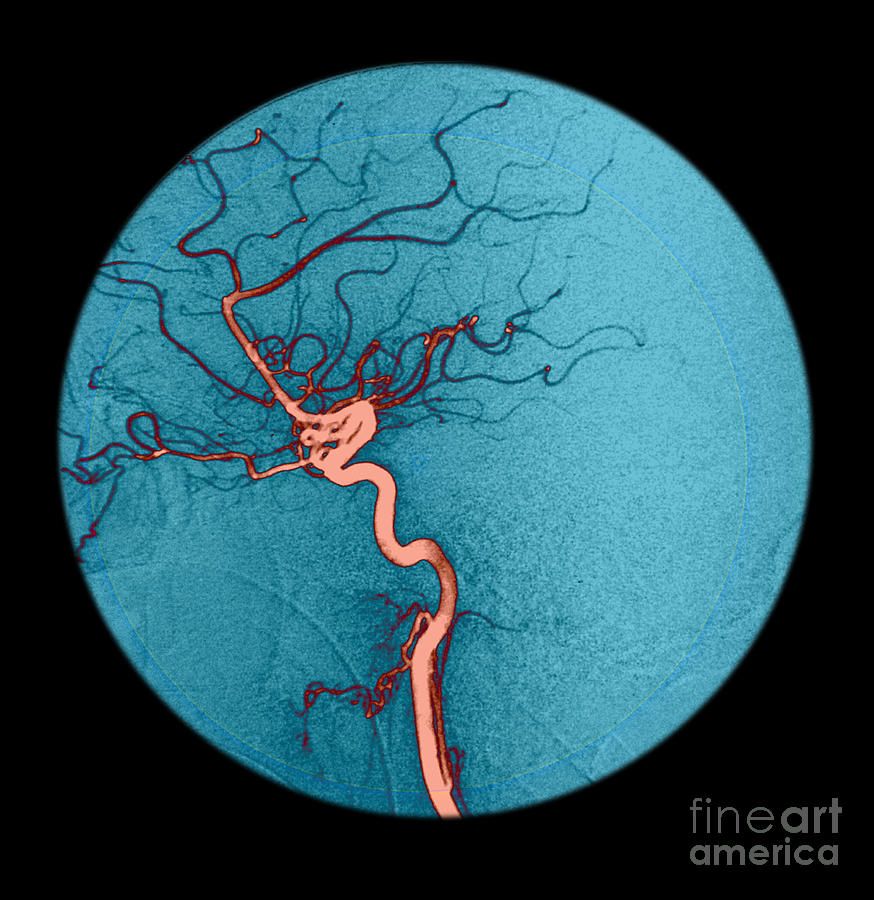This image from Fine Art America depicts a microscopic or highly magnified view centered on a perfect circle with a vivid, light blue background against a pitch-black square frame. The center of the circle is dominated by a thick, pinkish vein-like structure that branches out into numerous red squiggly lines, resembling the intricate network of veins or possibly even microorganisms. Interwoven among these red lines are black squiggly lines, creating a complex, interconnected pattern. Subtle green shading can be observed in parts of the blue area, adding depth to the image. The circle’s border and background are stark black, enhancing the vividness of the colors within. The image is signed "Fine Art America" in various fonts in the bottom right-hand corner.